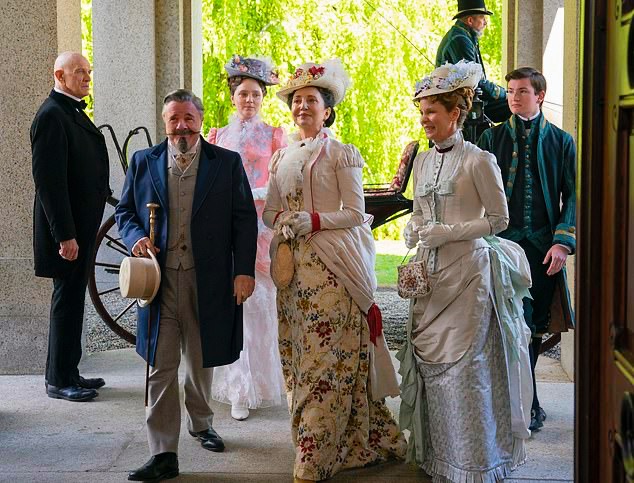In this detailed image, reminiscent of a scene from "Bridgerton," a group of people is captured standing in period clothing that showcases historic dress. At the forefront, three individuals immediately draw attention: a distinguished gentleman on the left, holding a cane in his right hand and wearing a beige suit with a blue jacket and a white top hat; next to him stands a woman adorned in a floral dress, holding a small cloth purse and wearing an ornate dressy hat; beside her is another elegantly dressed woman in a blue formal gown with a matching fancy light blue hat. These central figures are part of a larger group that includes three women, all in elaborate, ornate dresses and hats, and four men, showcasing a variety of distinguished period outfits.

To the left of the group stands a bald man in a long black coat with a bow tie, staring intently at the people; his demeanor and attire suggest he is a butler. Behind this main group, another man, possibly a servant, is also visible. He has gray hair, a mustache, and beard, and is dressed in a gray suit with a navy jacket, holding a hat and a cane.

In the background, the scene extends to a carriage setting where a man in livery is seated atop the vehicle, and another stands by, appearing to help escort the arriving party to a grand house entrance. This provides a glimpse into the elaborate process of their arrival, enhancing the historical authenticity of the scene.